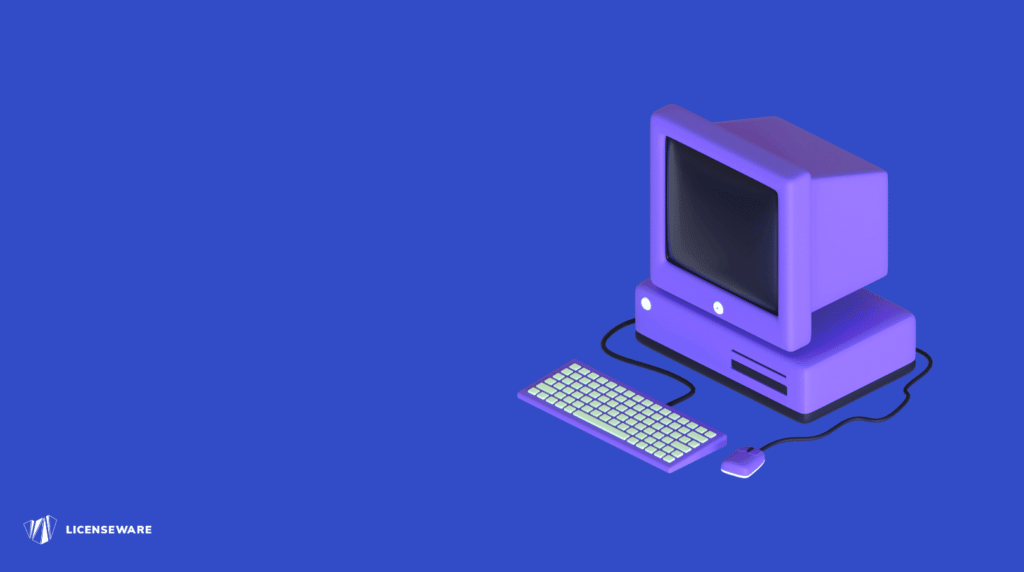In this image, a vintage computer model from the 80s or 90s is displayed prominently on the right side, facing left. Both the computer's outer case and the box it rests on are a striking purple color, and the monitor, which is currently off, has a black screen. Connected to the back of the computer are a matching purple mouse and keyboard, the latter featuring white keys. The monitor also features two white buttons. At the bottom part of the computer, there is an area to insert a CD. The background of the image is a blend of blue and purple hues. In the bottom left corner, the text "License Wear" is written in white next to a logo composed of three white shapes. This detailed illustration captures the nostalgic essence of older computer technology with modern graphical elements.